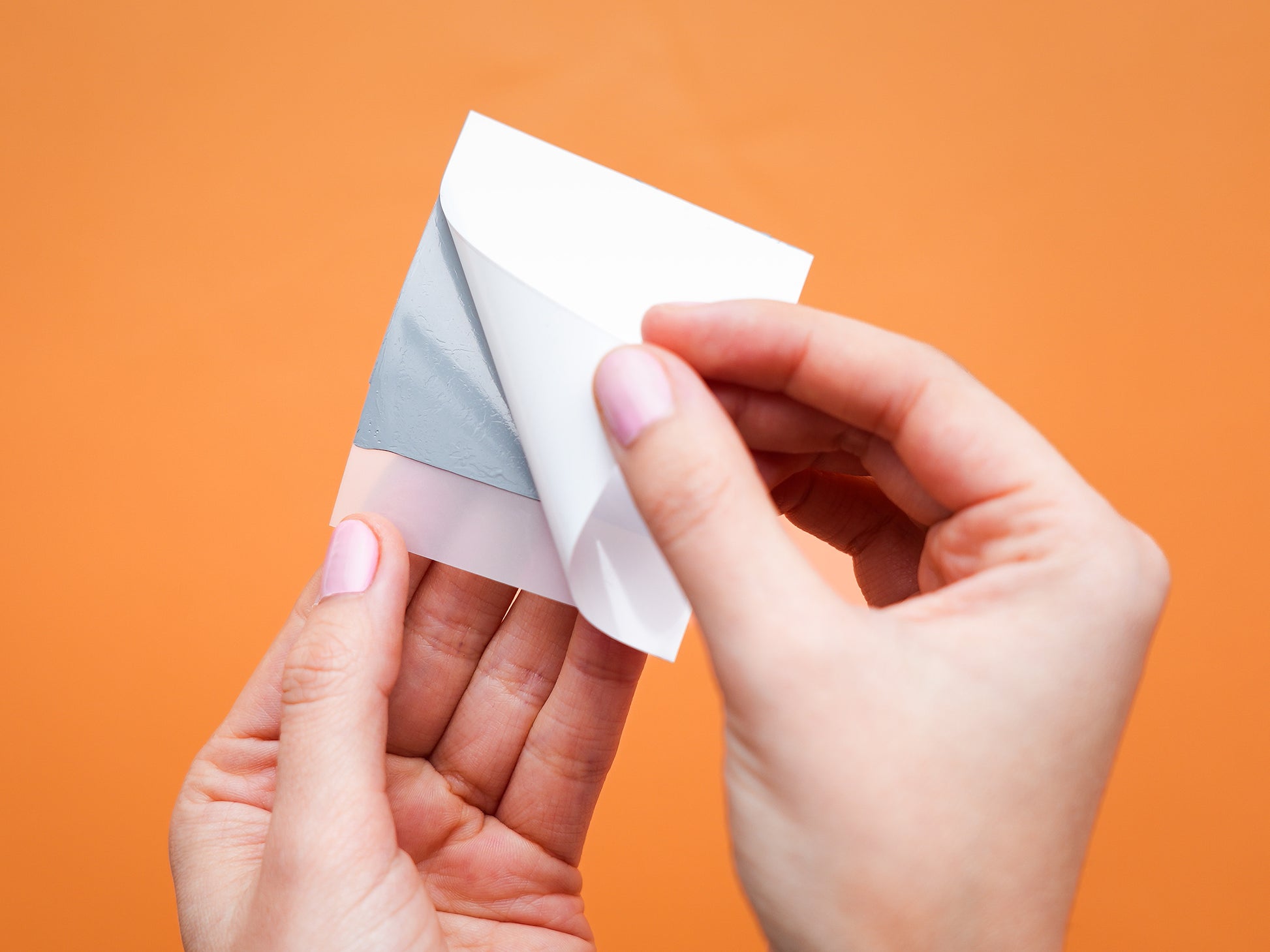In the image, two hands with pink nail polish are meticulously peeling back the adhesive layer of a square piece of glossy white sticker paper, revealing a clear backing with a notable gray stripe. The left hand secures the bottom left corner of the paper while the right hand lifts the adhesive layer from the same corner. Set against a bright orange background, the small, delicate sticker paper fits comfortably in the woman's hand, emphasizing both the product's compact nature and ease of use.